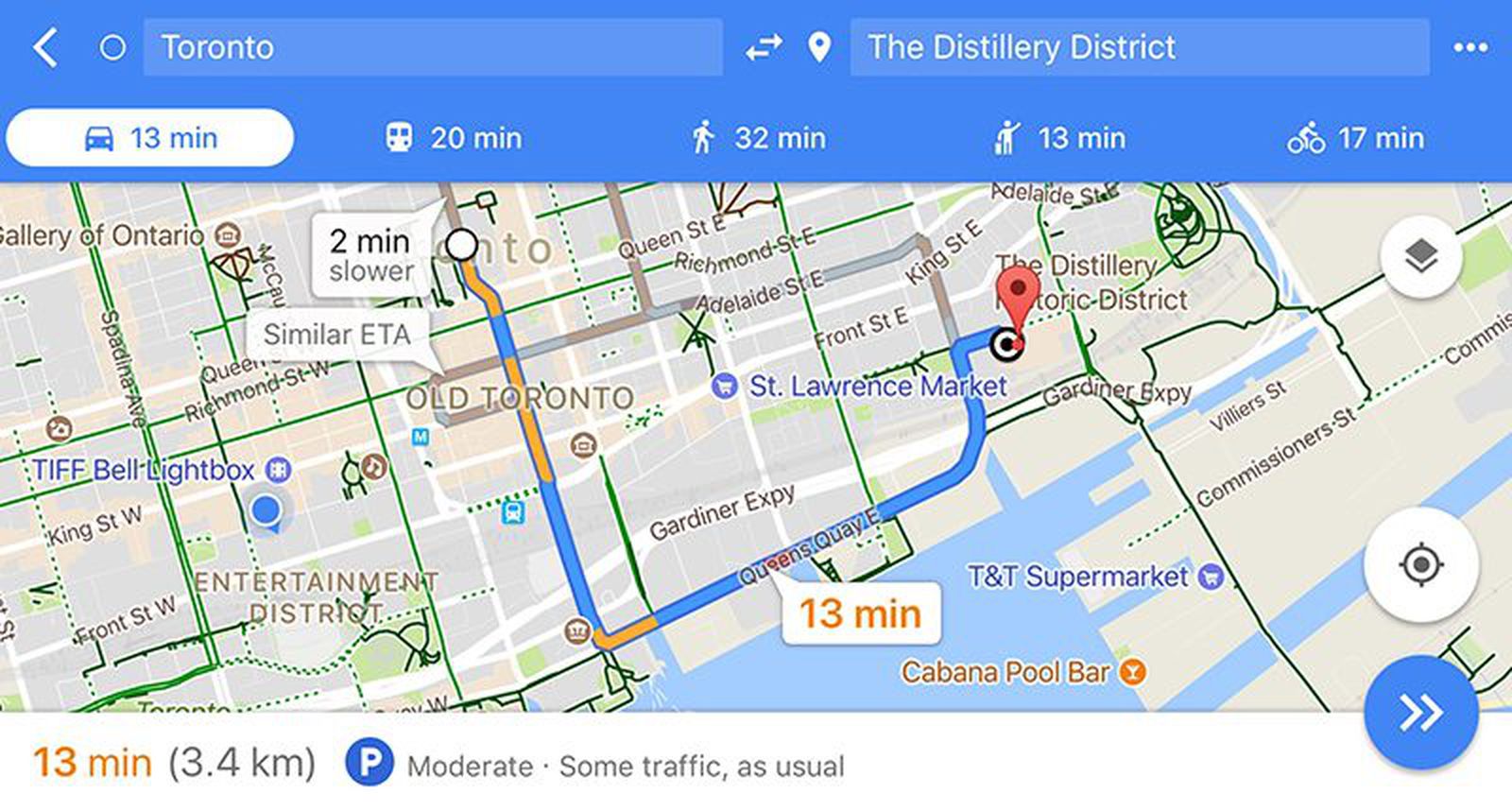**Descriptive Caption:**

A detailed screenshot of a map application, likely captured from a horizontally oriented device such as a tablet, displaying a segment of Toronto. The interface at the top features a blue bar with search boxes; in one of them, "Toronto" is typed, while the other suggests a destination, "Distillery District." Below this bar is the map itself, depicting a close-up of an area in Old Toronto.

The map predominantly uses a gray background, with streets highlighted in white and certain roads or areas marked in green. Notably, a box indicating "13 minutes" is present on the map, suggesting estimated travel time. Additionally, a  white speech bubble at the top also reads "13 minutes" next to a car icon, indicating driving directions.

A significant marker, represented by a large arrow, points to St. Lawrence Market, a known landmark in Toronto. At the bottom of the map, there is an annotation indicating moderate traffic conditions with a note of "traffic as usual." The overall presentation is clean and informative, serving as a navigational aid within the Old Toronto district.